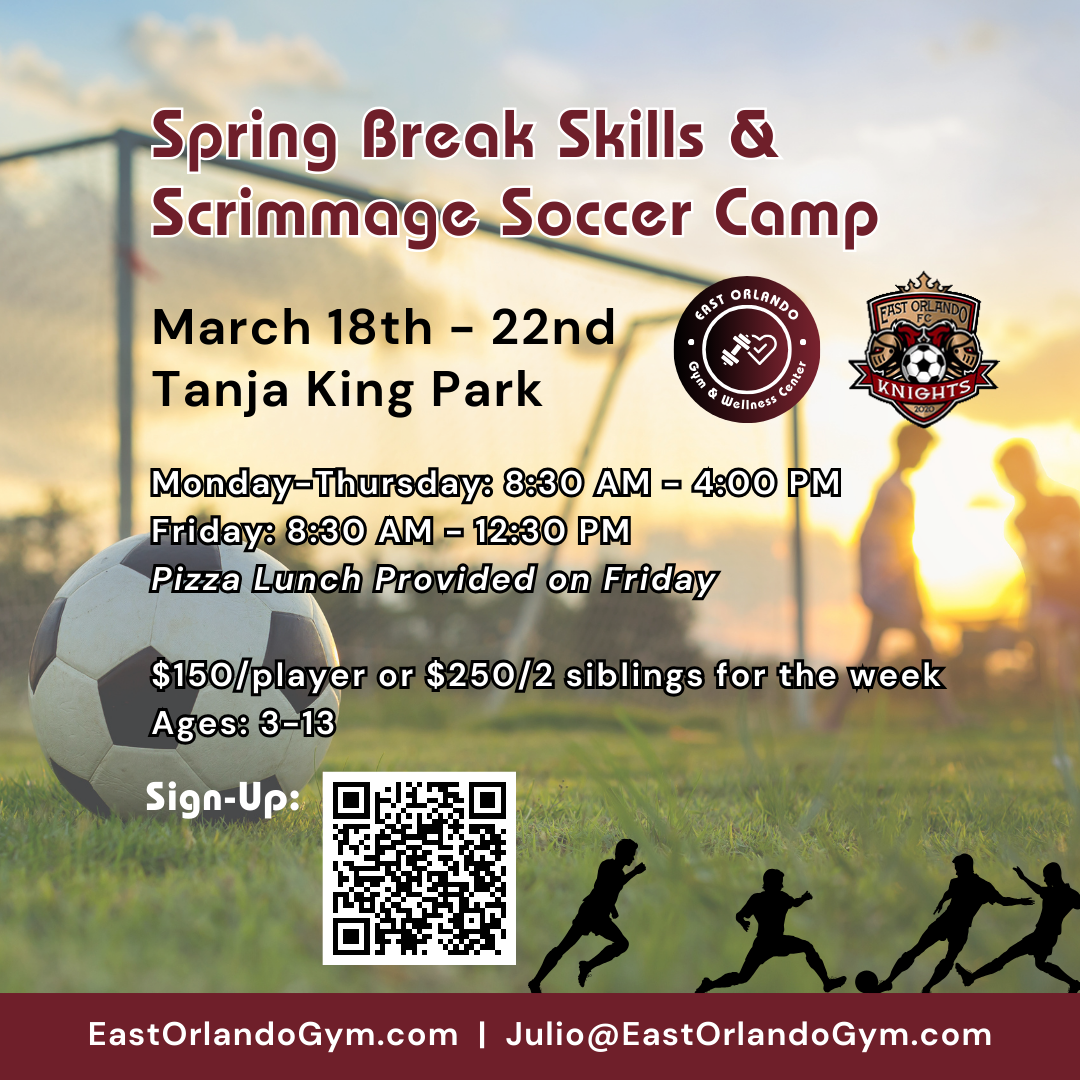The flyer is an advertisement for the "Spring Break Skills and Scrimmage Soccer Camp," emphasized by maroon, sans-serif text with a white outline at the top. This event is scheduled from March 18th to 22nd at Tanja King Park. Key details include the camp operating Monday to Thursday from 8:30 a.m. to 4:00 p.m., and Friday from 8:30 a.m. to 12:30 p.m., with a pizza lunch provided on Friday. The cost is $150 per player or $250 for two siblings for the week, catering to children aged 3 to 13. Essential information, such as sign-up details, is illustrated through a QR code at the bottom, accompanied by contact info in a red rectangle: eastorlandogym.com and julio@eastorlandogym.com.

The flyer features overarching green hues, interspersed with sunset-colored silhouettes of players vying for a ball, and a central black and white soccer ball. A goal post marks the center background, while the right side showcases logos for East Orlando Gym and First Orlando FC Knights, each within dark red circles highlighting a dumbbell-heart combo and knights in armor. The bottom right is adorned with more silhouettes of playing teens, creating a dynamic and sporty ambiance.